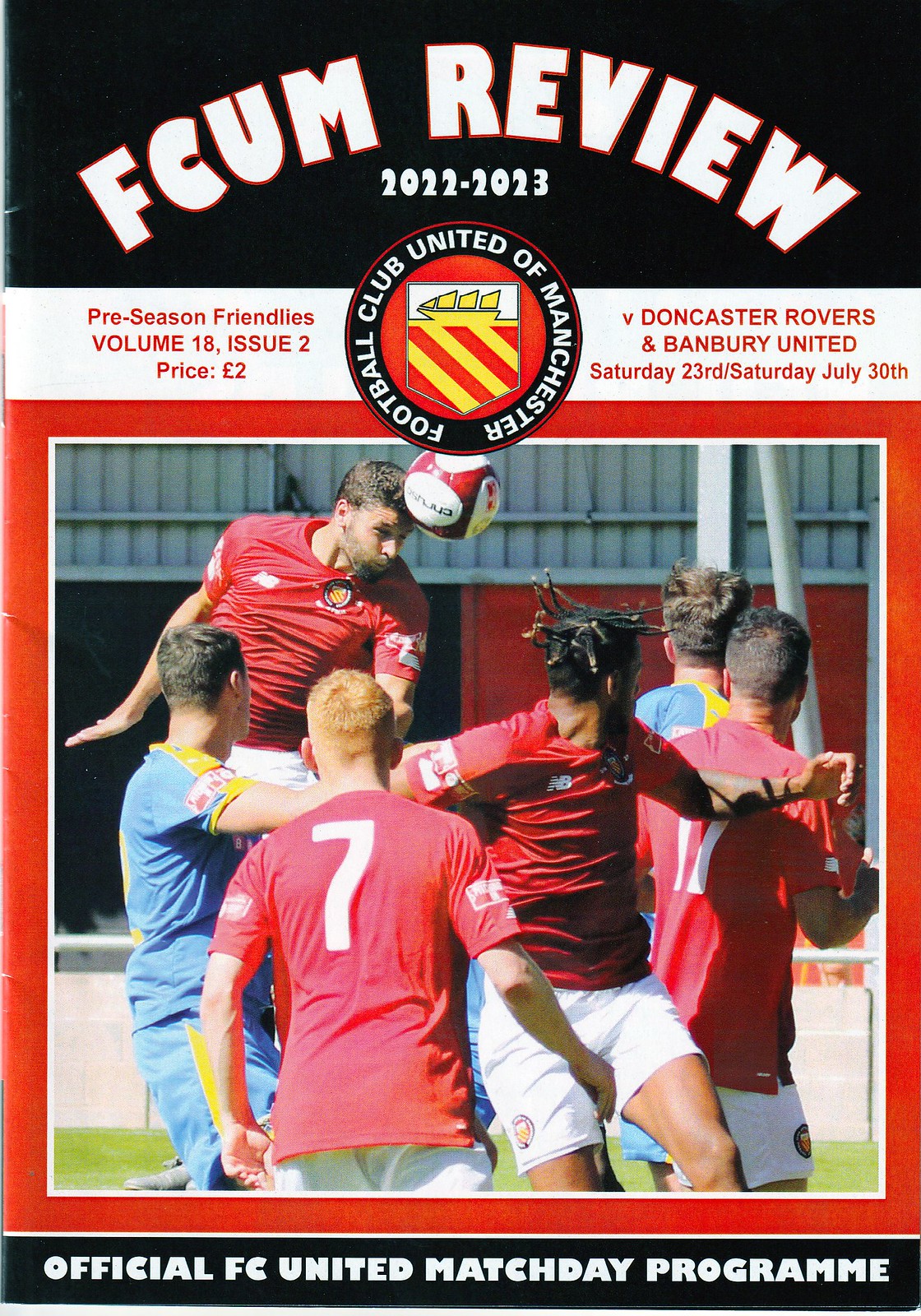This image is the cover of an official matchday program for Football Club United of Manchester, titled "FCUM Review 2022-2023." At the top of the cover, within a black rectangle with white text outlined in red, it reads "FCUM Review 2022 to 2023." Just below this, a white banner features the club's logo: a black circle with a red circular border and a shield crest in the center. The shield boasts diagonal red and yellow stripes and a stylized yellow ship at the top. 

On the left side of the banner, in red font, it reads "Preseason Friendlies, Volume 18, Issue 2, Price £2." On the right side, it lists "Doncaster Rovers and Banbury United," along with their match dates, "Saturday 23rd, Saturday July 30th." Below the banner, framed in red, is a dynamic photograph capturing a soccer game. 

The image prominently features a player in a red shirt heading the ball, with other players visible in varying stages of motion. Four of the players are in red shirts and white shorts, while two others wear blue and yellow shirts. At the bottom of the cover, within a black border, the text reads, "Official FC United Matchday Program."